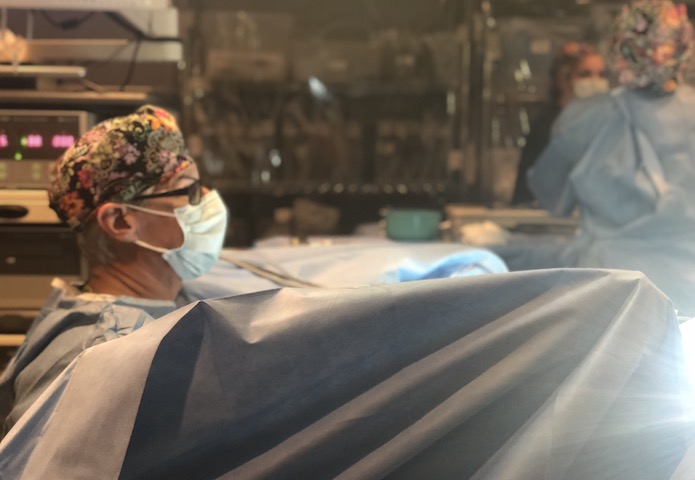The image depicts the interior of a surgical room. Dominating the left side of the picture is the profile of a focused medical professional, clad in a blue paper gown and a blue mask. This individual also wears black-framed glasses and a multicolored, floral-patterned surgical cap. Their hands, also in blue paper coverings, extend to the right of the frame. Behind this person, various pieces of medical equipment are visible, including machines with digital readouts and shelves stocking surgical supplies. The right side of the image shows two more masked and scrub-clad medical professionals, also wearing head coverings. A gray plastic tarp occupies the lower portion of the image, partially obscuring the scene and hinting at an ongoing surgical procedure. Bathed in a soft light emanating from the right side, the entire scene is imbued with the sterile, clinical ambiance typical of an operating room.